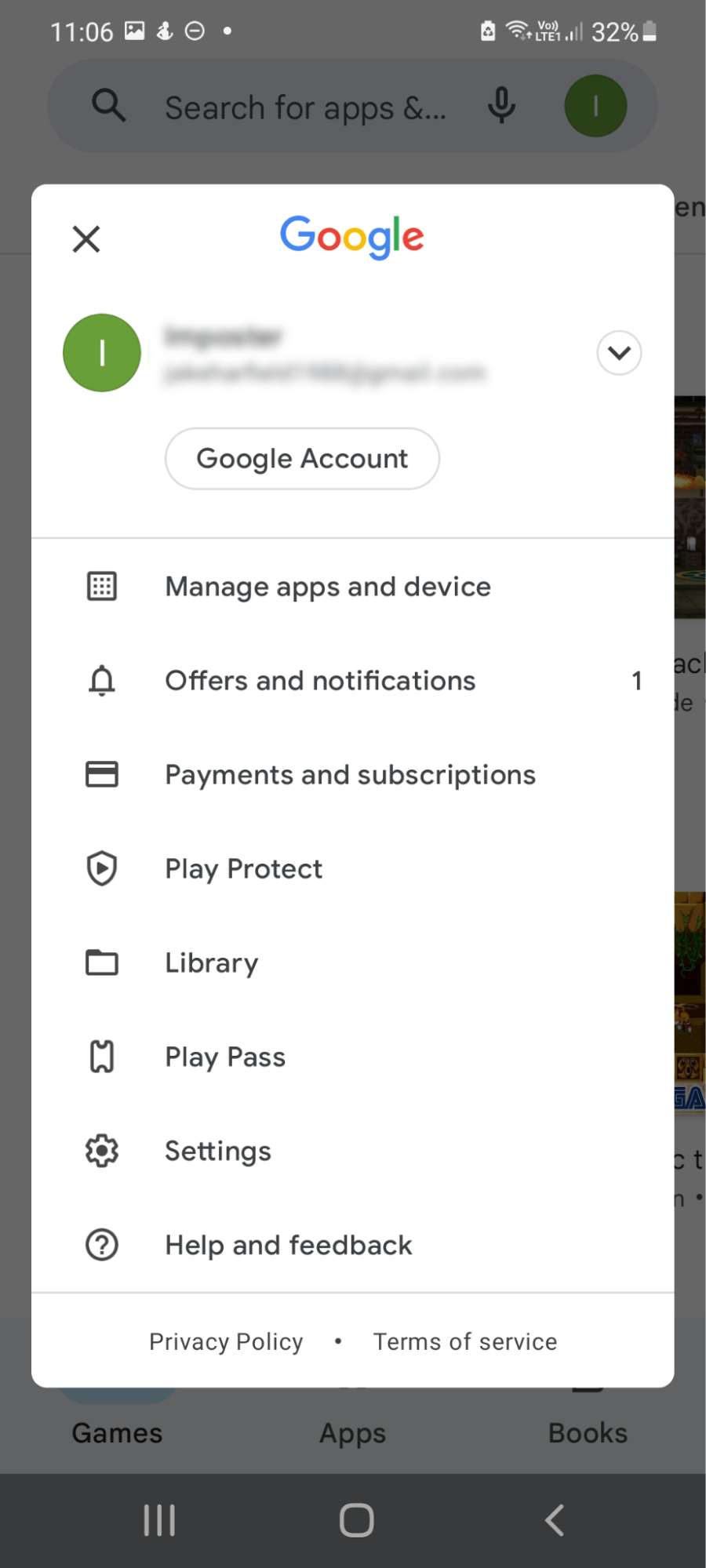The image depicts a smartphone screen, with the time showing 11:06 and the battery level at 32%. At the top of the screen, there is a search bar featuring a magnifying glass icon, a microphone icon, and the text "Search for apps." Below this bar, there's a prominent section with the Google logo, which features the blue, red, yellow, and green colors. Next to the logo is a close button (X) on the left and a green oval with the number "1" in it. 

Directly below these elements is the text "Google account" accompanied by a drop-down arrow. Following this, several options are listed: "Manage apps and devices," a bell icon (offers and notifications) marked with a number "1," a credit card symbol (payment and subscriptions), a shield with a play button (Play Protect), a file icon (Library), a puzzle piece icon (Play Pass), and a gear icon (Settings). Further down, there is a question mark inside a circle labeled "Help & feedback."

A horizontal line separates these sections from the final set of options, which include "Privacy Policy," "Terms of Service," and categories like "Games," "Apps," and "Books." At the very bottom of the screen are three lines (menu button), a stop button, and a reverse button.